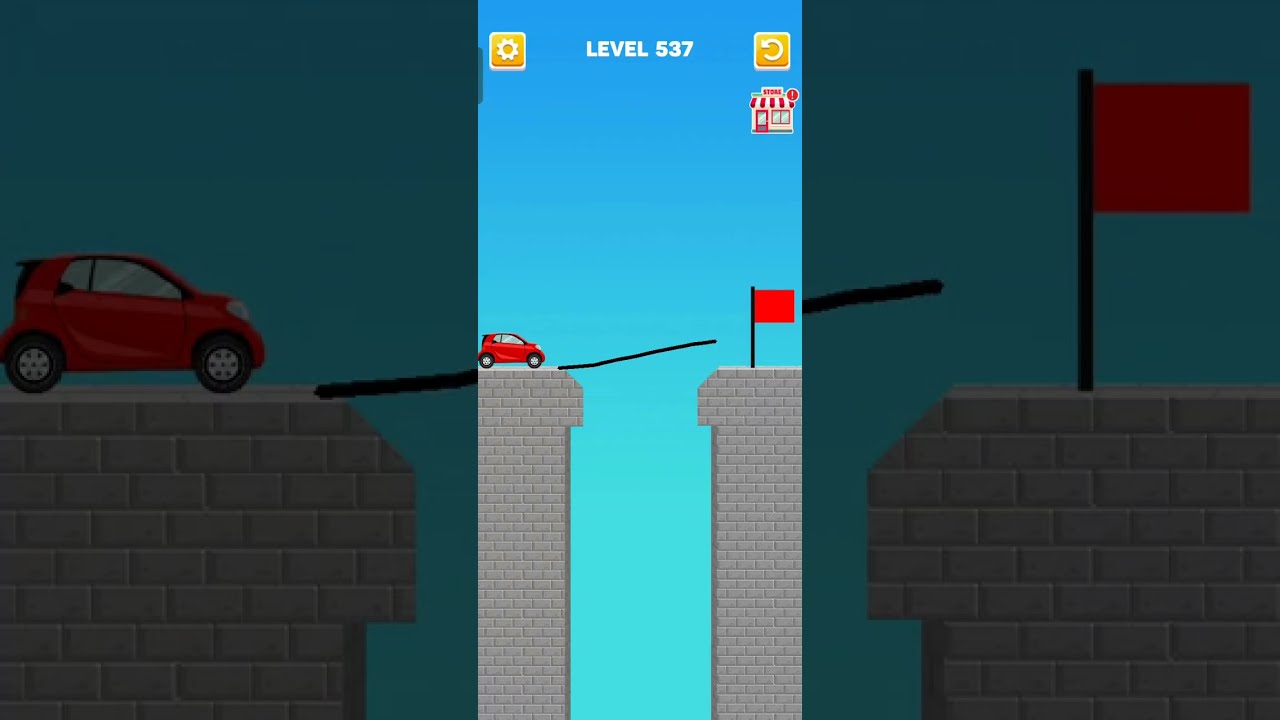The image depicts a screenshot from a mobile game app in a portrait orientation, featuring a central gameplay scene framed by two grayed-out side bars. The main game screen shows a small red car poised to jump over a gap between two tall, gray brick towers. On the left tower, there's a red car, and on the right tower stands a black flagpole with a red flag. A thin black line spans the gap, indicating a path the car must take, suggesting a physics-based challenge. At the top of the screen, the text "Level 537" appears in white on a blue background. In the upper left corner, there is a yellow square with a white settings cog, while the upper right corner features a yellow square with a white return arrow. Below the return button, a small white and red shop icon is visible. The background of the entire image is blue, reinforcing the impression that the scene is set outdoors in a stylized, animated environment.